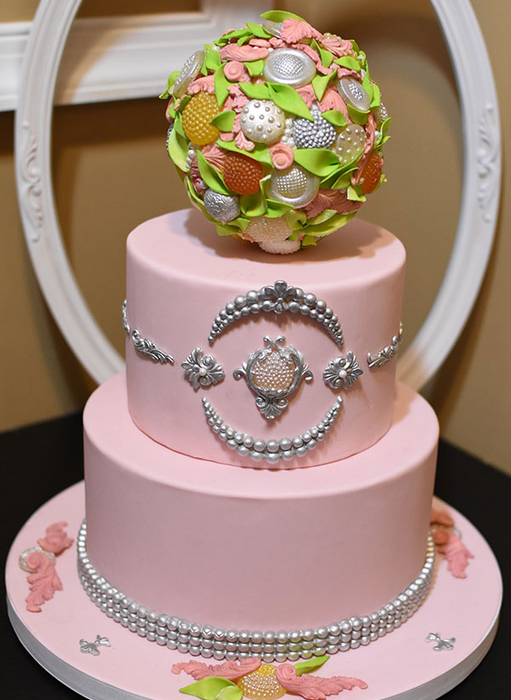Displayed on a black table, the image showcases a stunning, ornate wedding cake set against a tan-colored wall. The backdrop features a white, oval-shaped frame at the top edge, adding a classic touch to the setting. This three-layer cake, primarily pink in color, appears to be made of fondant. Each tier of the cake is smaller than the one below it, creating a tiered structure. The base is adorned with three stacked rows of silver pearls encircling the bottom layer. The second layer features a silver emblem resembling a flower bouquet, accented with additional silver decorations. Crowning the top layer is a spherical ornament composed of small silver balls, resembling an intricate ball of fabric roses with pink flowers and green leaves embedded within.